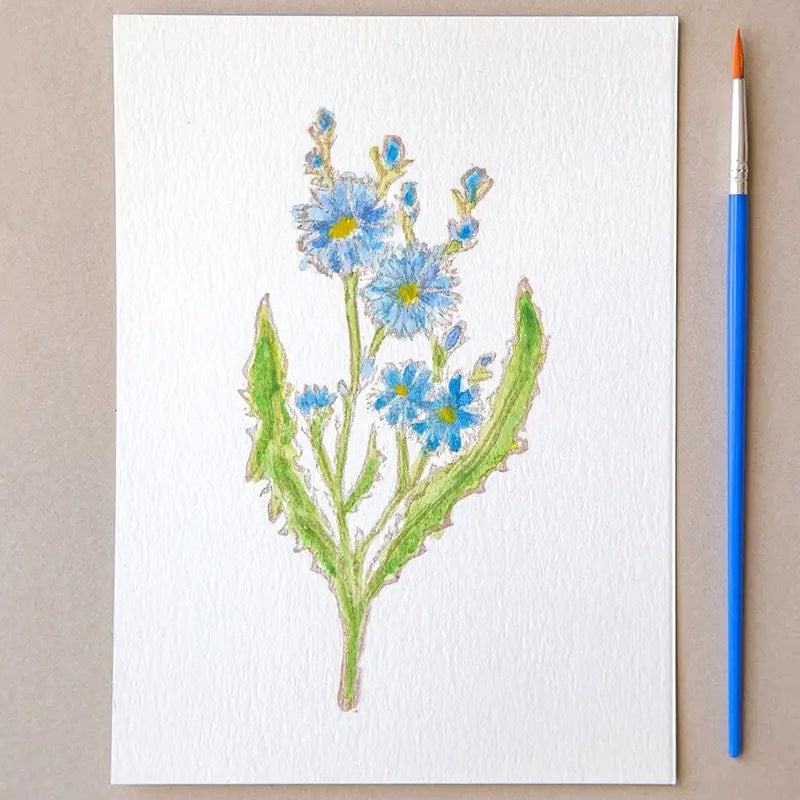This image showcases a detailed watercolor painting of delicate flowers. The artwork is composed on a white, thick rectangular sheet of paper that lies on a light gray table against a beige background. To the right of the paper, there is a light blue paintbrush with a fine point and an orange bristle tip, featuring a thin silver metal ferrule. The painting itself depicts a plant with a gray outline at the base, branching out into stems and leaves colored in light green. The stems support a collection of blooming flowers with baby blue petals and vibrant yellow centers. There are five prominent flowers visible, accompanied by additional buds beginning to emerge at the top. The composition illustrates the beauty of nature through the fine details and soft color palette of the watercolor medium.